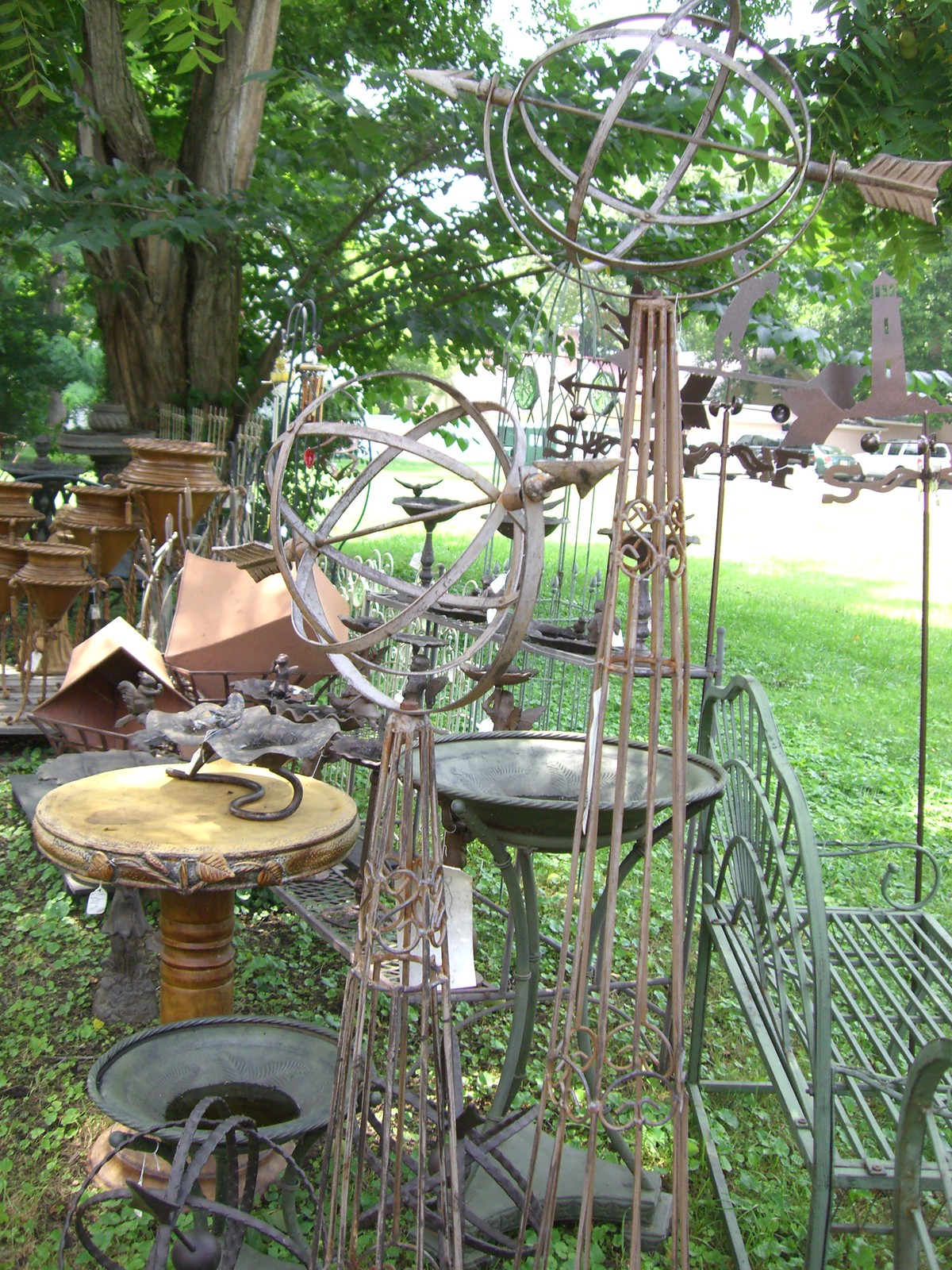This photograph captures a vibrant outdoor display featuring an eclectic collection of yard ornaments and wrought iron sculptures, set against a lush, green grassy area. A dominant mature tree with a uniquely three-trunked base and a rich canopy of green leaves stands in the upper left corner, partially framing the scene. Below the tree, four brass vases are arranged systematically, contributing to the decorative appeal. The main focus of the image is a clustered arrangement of various outdoor decorations, including a grayish-green metal bench positioned in the lower right corner and three ornately designed birdbaths. One birdbath features a black iron pedestal and a scalloped basin adorned with a detailed bird sculpture. Adjacent to these, two windmill-like metal structures with intricate designs act as ornamental wind catchers. Additional whimsical items, such as a small metal bull and other unique metal artifacts, populate the background, enhancing the charm and eclectic nature of the setting. The road, barely visible in the upper left section of the photograph, hints that this lively display may be part of someone’s front yard.